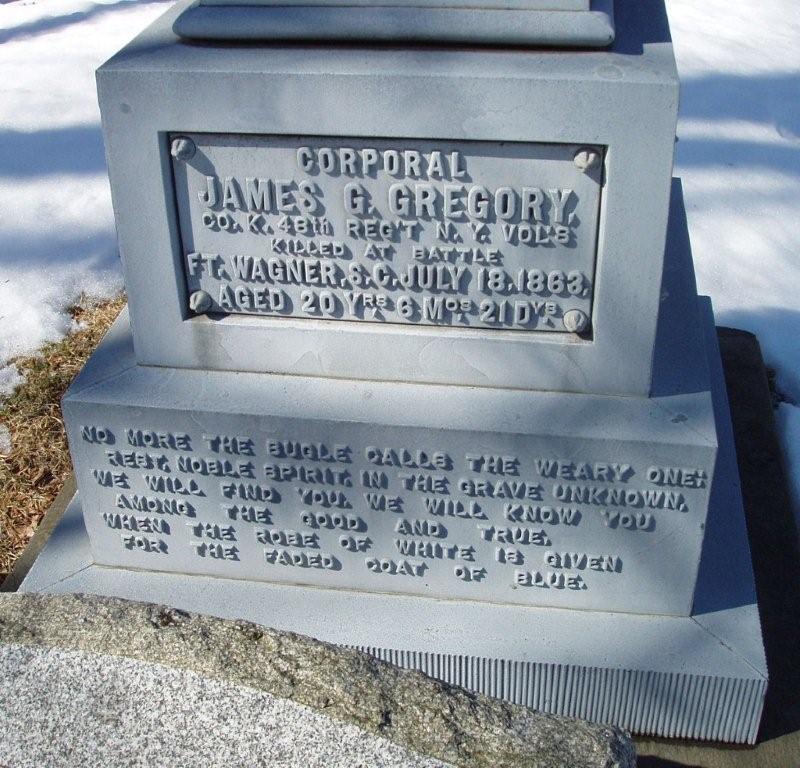The image depicts a three-tiered granite memorial stone partially covered in snow, with patches of grass visible to the side. At the monument's base, there is a blue-gray square, which supports a larger stone block, followed by a smaller block on top. The inscription on the stone honors Corporal James G. Gregory of Company K, 48th Regiment, New York Volunteers, who was killed at the Battle of Fort Wagner, South Carolina, on July 18, 1863, at the age of 20 years, 6 months, and 21 days. Below the main inscription, a poignant epitaph reads: "No more the bugle calls the weary one, rest noble spirit in the grave unknown. We will find you, we will know you among the good and true when the robe of white is given for the faded coat of blue."